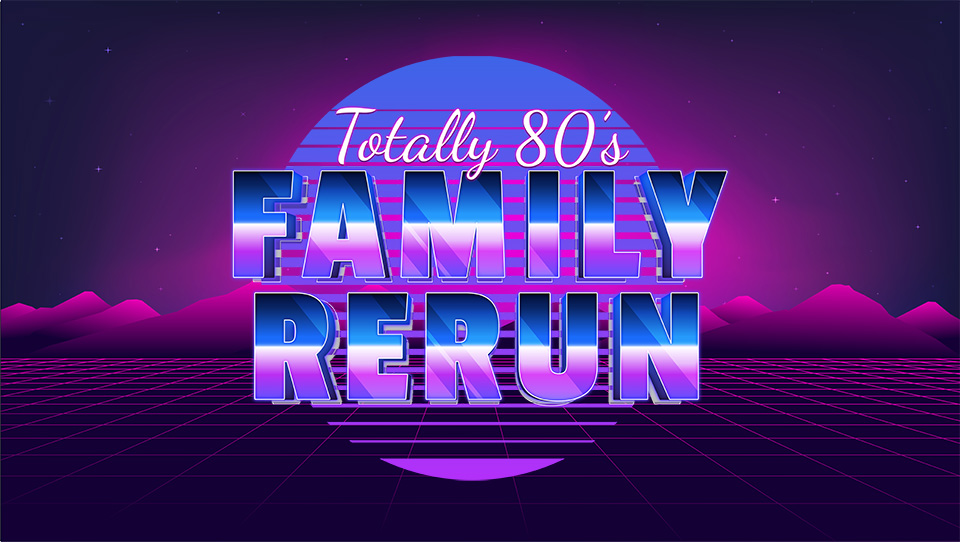The image showcases a vibrant, retro-esque style logo rendered in the popular Vaporwave aesthetic. Dominated by grid-based, almost 3D-like elements, it bursts with metallic neon colors. The background features striking 2D mountains, predominantly black at the bottom, seamlessly transitioning into pink hues. The lower half of the image is characterized by an intricate pink grid landscape. Above, a dark sky speckled with pink stars sets a moody yet sparkling ambiance. At the heart of the logo lies a central purple circle, segmented horizontally by multiple pink lines. This circle encapsulates the text “Totally 80s Family Rerun,” with the phrase “Totally 80s” inscribed in a cursive white font and “Family Rerun” employing a gradient palette transitioning from dark blue to white to purple. The overall design masterfully blends nostalgic 80s elements with modern artistic flair, evoking a sense of animated, almost cartoonish nostalgia.